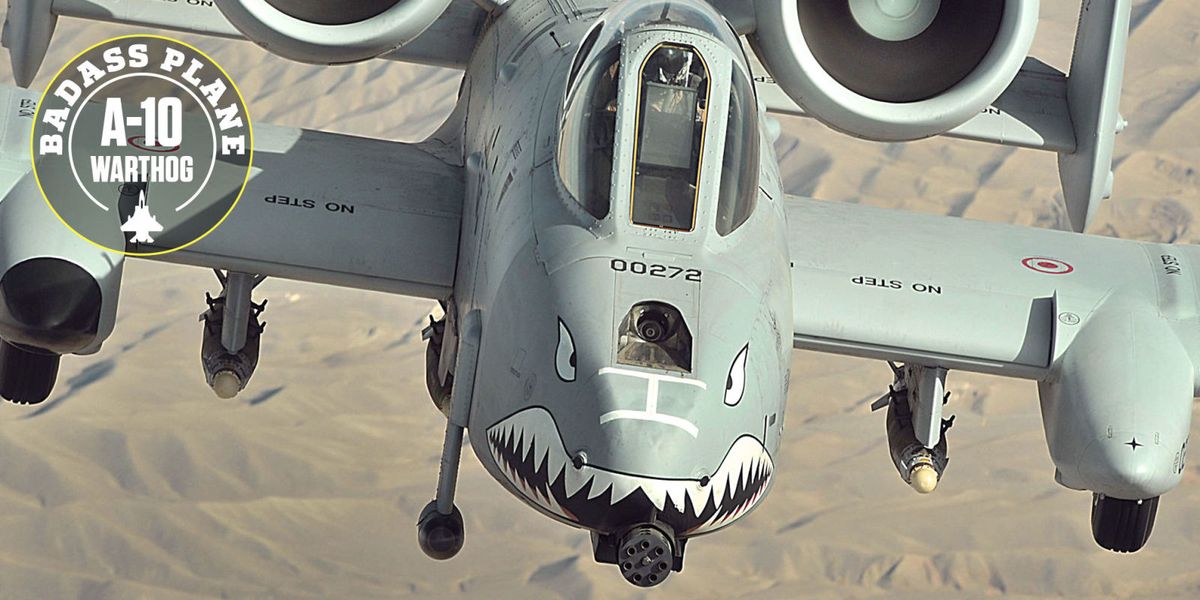This detailed image captures an A-10 Warthog warplane, as indicated by the "badass plane A-10 Warthog" emblem in the upper left corner, accompanied by a small symbol of a fighter jet. The plane's body is primarily light army green with gray sides, and its striking front features a fierce, shark-like face adorned with eyes, a mouth full of teeth, and a nose, reminiscent of a warthog. The nose also houses a Vulcan minigun, with a radar pole extending from it. Each wing of the Warthog showcases red bullseye targets and the words "NO STEP" in the corners. Notably, the plane is equipped with missiles under each wing and one beneath its belly. Two turbine engines are mounted on the top back portion, just behind the glass pilot pod, where the helmeted pilot is visible. The plane is flying over a desert landscape, and on its top side, the numbers "00272" are displayed.